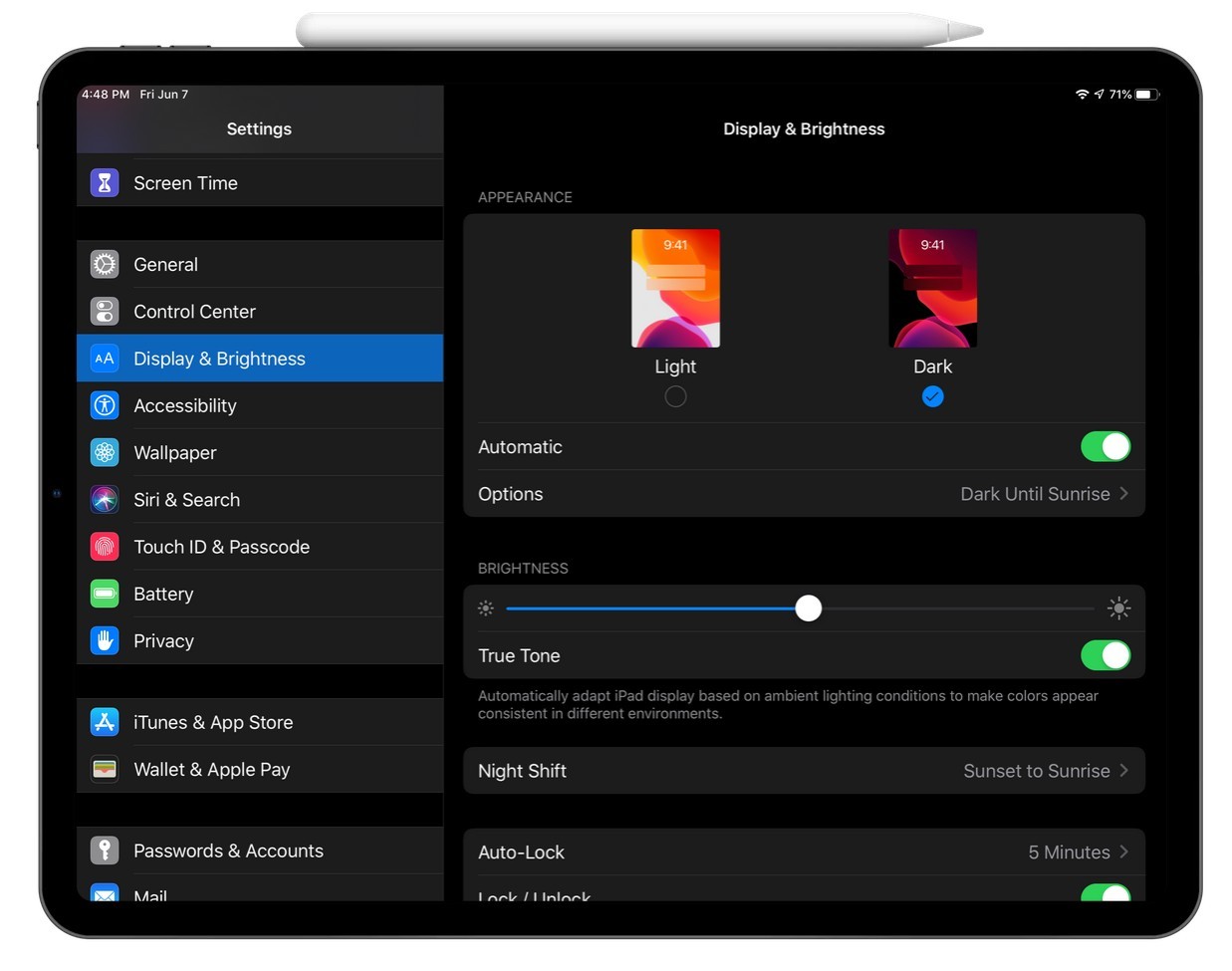A detailed image of a black tablet with visible edges and a white stylus resting on the top. The screen displays a settings menu with the following details: 

- **Top left corner:** 4:48 p.m., Friday, June 7
- **Left sidebar options:** Settings, Screen Time, General, Control Center, Display & Brightness, Accessibility, Wallpaper, Siri & Search, Touch ID & Passcode, Battery, Privacy, iTunes & App Store, Wallet & Apple Pay, Passwords & Accounts, Mail
- **Main screen background:** Blue with white text highlighting "Display & Brightness"
- **Main screen title:** Display & Brightness
- **Appearance settings:** 
  - Light
  - Dark (checked)
  - Automatic (toggled on, green)
  - Options include: Dark until sunrise
- **Brightness setting:** A blue and gray slider positioned in the middle
- **True Tone:** Toggled on (green). The description reads: "True Tone automatically adapts iPad display based on ambient lighting conditions to make colors appear consistent in different environments."
- **Night Shift:** Set from Sunset to Sunrise, indicated by a right arrow
- **Auto-Lock settings**